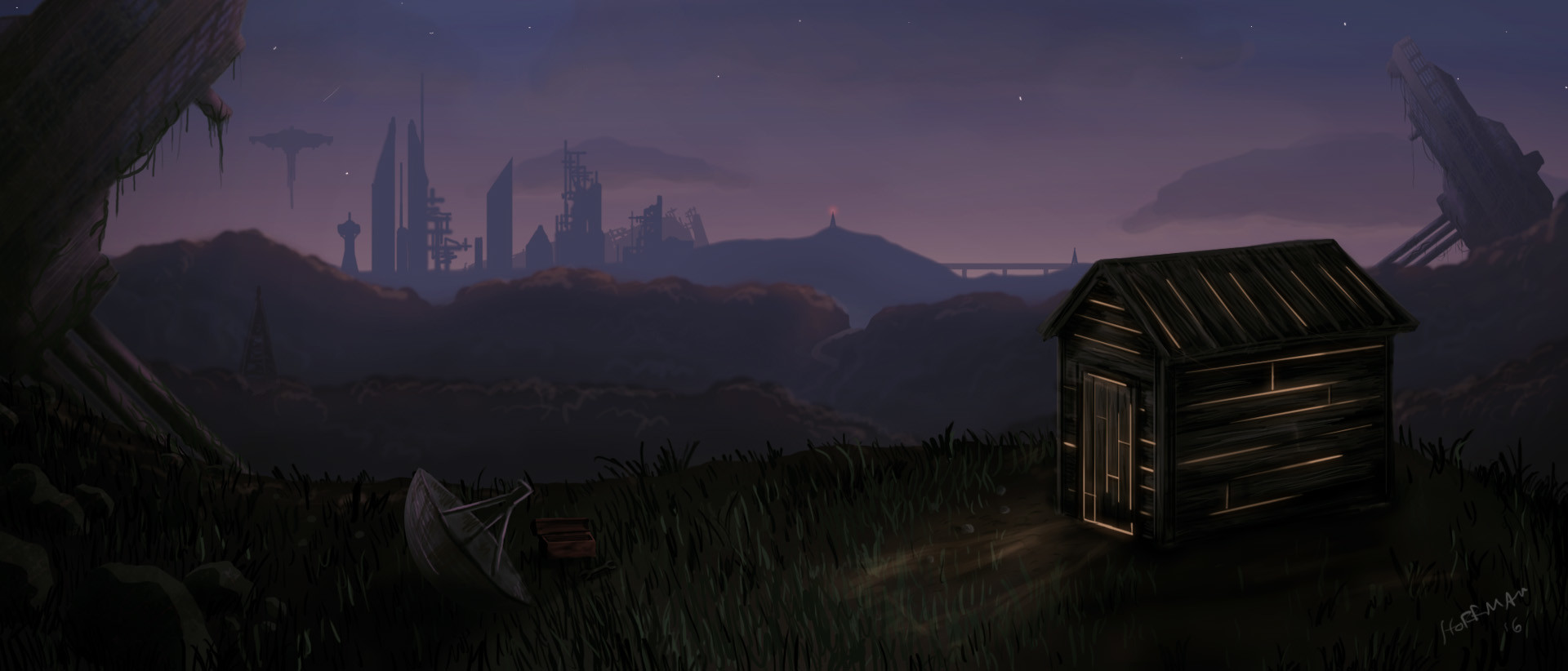This digital artwork, possibly created using computer-generated techniques, depicts a serene nighttime scene in a wilderness setting. The image, rectangular in shape and measuring approximately 5 inches wide by 2 inches high, features a small wooden cabin situated on top of a grassy hill. The side view of the cabin reveals an amber light glowing from within, casting a warm and inviting ambiance. To the left of the cabin lies a broken satellite dish, adding a touch of intrigue. Beyond the hill, a range of additional hills stretches into the distance, leading to the dark grey silhouettes of large buildings. The sky above is a dark, deep blue or purple, speckled with white dots representing stars and partially covered with clouds. The upper half of the image also includes tall cylindrical buildings and floating structures on the left, with a lighthouse and a bridge visible in the center and to the right. In the bottom right corner of the image, the artist's name, "Hoffman," is inscribed in Blueprint, accompanied by the number "6." The overall atmosphere is one of quiet isolation, accentuated by the remote, poorly lit landscape.